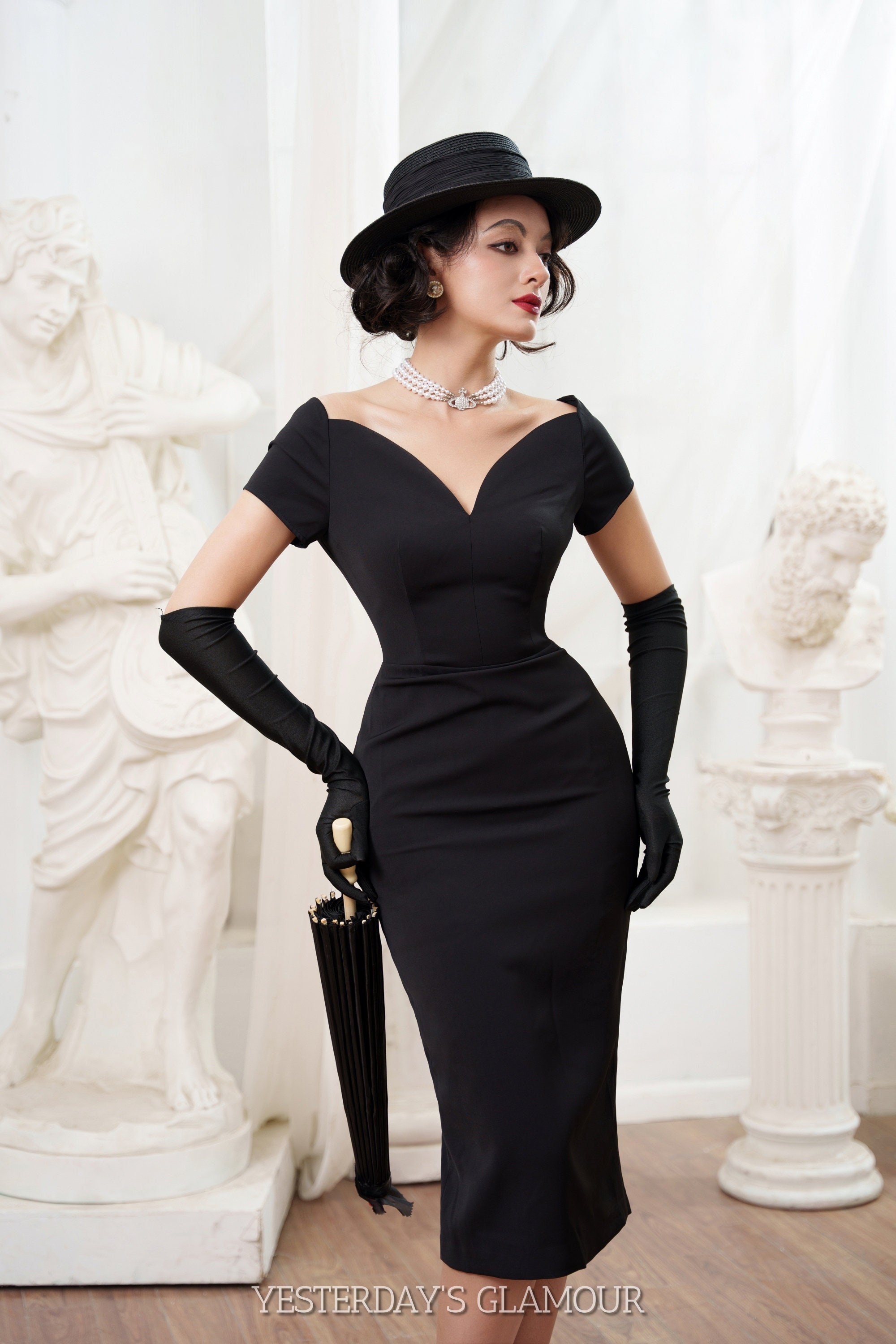The color photograph captures a styled young woman in a museum-like setting, styled in classic vintage fashion reminiscent of the 1950s to 1970s. She is wearing a form-fitting, elegant black dress with a V-shaped neckline and short sleeves, accessorized with long black gloves that extend past her elbows. Her ensemble is complemented by a black round hat and a multi-layered pearl necklace, highlighted by a large central pearl. Her medium-length black hair and striking red lipstick add to her glamorous appearance. The black umbrella with a brown handle that she's holding in her right hand (left side of the image) adds a touch of sophistication. The backdrop features two statues: on her left, a bust of a bearded man on a pedestal, and on her right, a full-body statue of a man plucking a stringed instrument resembling a mandolin. The background behind these statues is a white curtain, with wood-paneling on the floor and an overhead light casting a soft illumination. At the bottom of the image, the caption reads "Yesterday's Glamour," anchoring the retro styling of the scene.